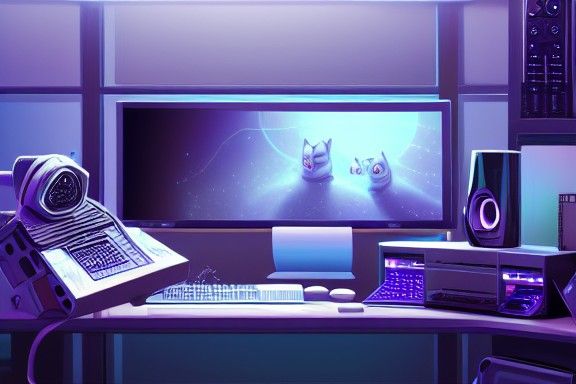The image appears to be an AI-generated or digitally illustrated scene of a high-tech office setup, bathed in purplish-blue and black hues. Dominating the scene is a curved desk stretching from left to right with a massive, elongated computer monitor mounted on the wall in front of it. The monitor displays an enigmatic image featuring two small, possibly owl or cat-like figures standing in front of a glowing orb of light, suggestive of a celestial or outer space setting.

Situated on the desk are multiple keyboards and a mouse. On the right side, there is a prominent disk drive section topped with a large speaker. To the left, a piece of furniture or control box with metal parts and buttons, possibly a defibrillator, stands tall, also featuring what seems to be a camera. On the upper right wall, a circuit board adorned with various knobs and buttons adds to the high-tech ambience. The entire scene, with its artistic and detailed composition, emits a vibrant, futuristic vibe.